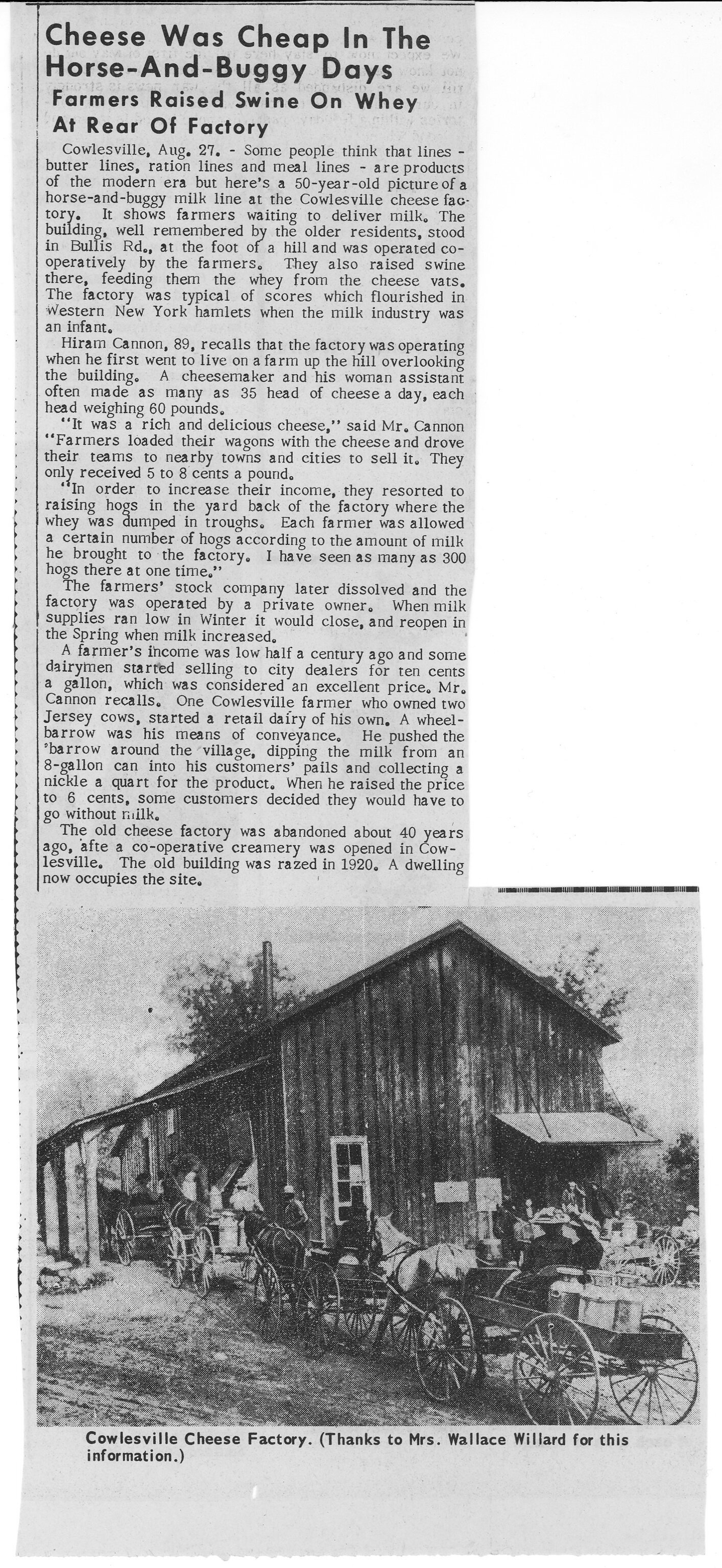The image presents a newspaper cutting adhered to a white surface, featuring a historical article entitled "Cheese Was Cheap in the Horse and Buggy Days: Farmers Raised Swine on Whey at Rear of Factory". Below the title is an extensive article exploring the Cowlesville Cheese Factory's history and its operations in the early 20th century. The detailed text vividly describes how farmers delivered milk by horse and buggy, with the factory's cheesemakers producing up to 35 hefty, 60-pound cheese wheels each day. Farmers earned just 5 to 8 cents per pound of cheese, prompting them to supplement their incomes by raising swine, who were fed whey leftovers from the cheese-making process. The article ©oncludes with a nostalgic recount of the factory's closure and the demolition of its wooden building in 1920.

Accompanying the article, at the bottom of the clipping, is a black-and-white photograph depicting the Cowlesville Cheese Factory. The image showcases an old wooden building with two eaves and several horse-drawn carriages lined up outside. The photo is captioned, "Cowlesville Cheese Factory. Thanks to Mrs. Wallace Willard for this information." This photograph and article together illustrate a vivid portrait of life and industry in Cowlesville during the horse and buggy era.